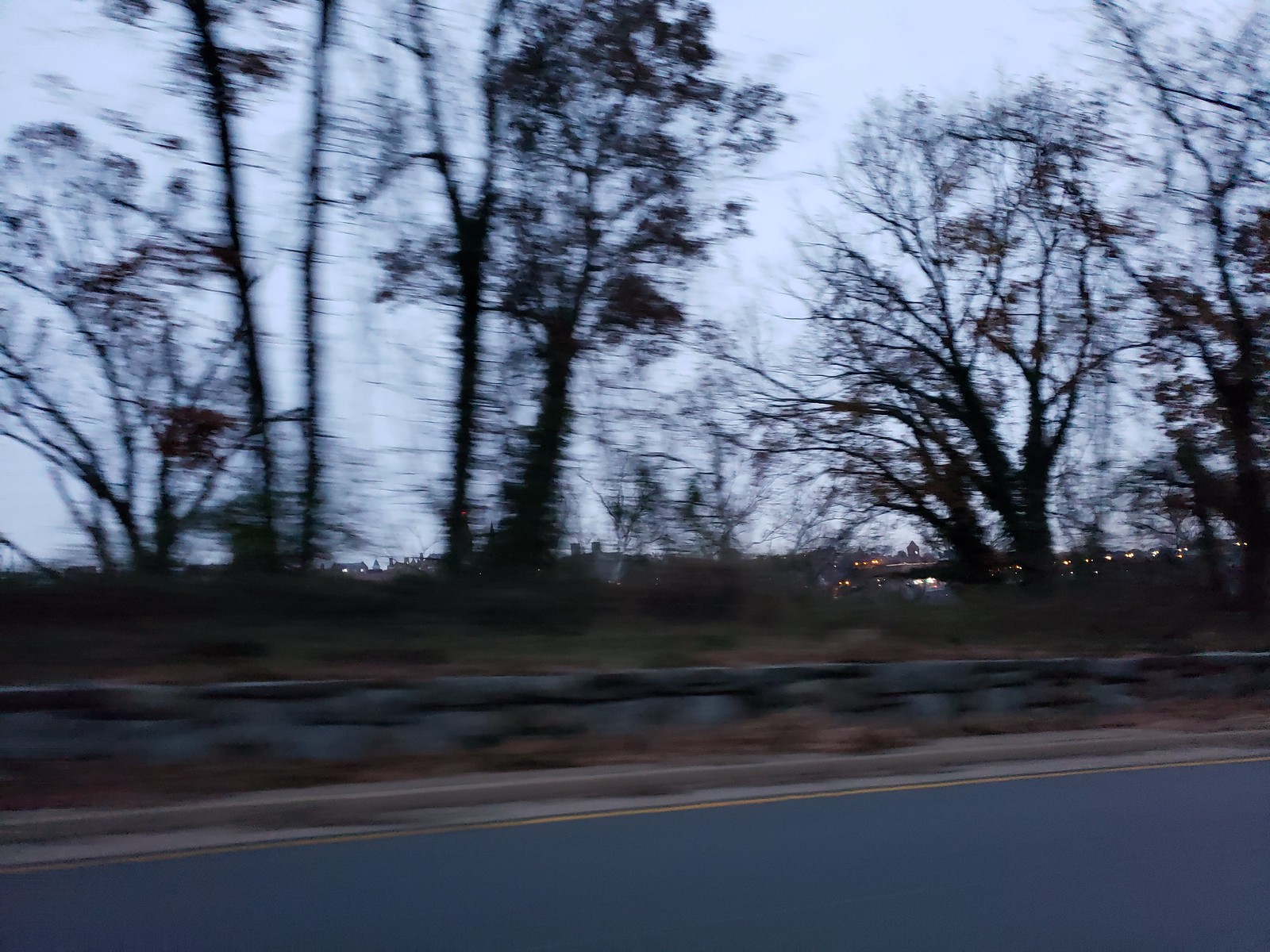This blurry photograph, likely taken from a moving vehicle at twilight, depicts an outdoor scene with multiple layers of interest. At the bottom of the frame, there is a smooth grey asphalt road marked by a thin yellow line near the edge. Adjacent to the road is a light grey to very light beige sidewalk covered with a stretch of dead brown leaves, which have accumulated against a partition or retaining wall made of large grey stones. Above the retaining wall is a gentle grassy slope interspersed with some brown patches and a line of shrubs. Further up the slope, a range of silhouetted trees of various shapes and sizes, some barren and some with few leaves, stand stark against the backdrop. Vines are noticeable on some of these trees. In the distance, on the horizon, there is a town or cluster of buildings with lit windows emitting colors from orangish-yellow to white. These buildings, mostly one or two stories high, shimmer faintly behind the silhouetted trees. The entire scene is enveloped by a solid grey sky, adding to the overall dusky, indistinct atmosphere of the photograph.